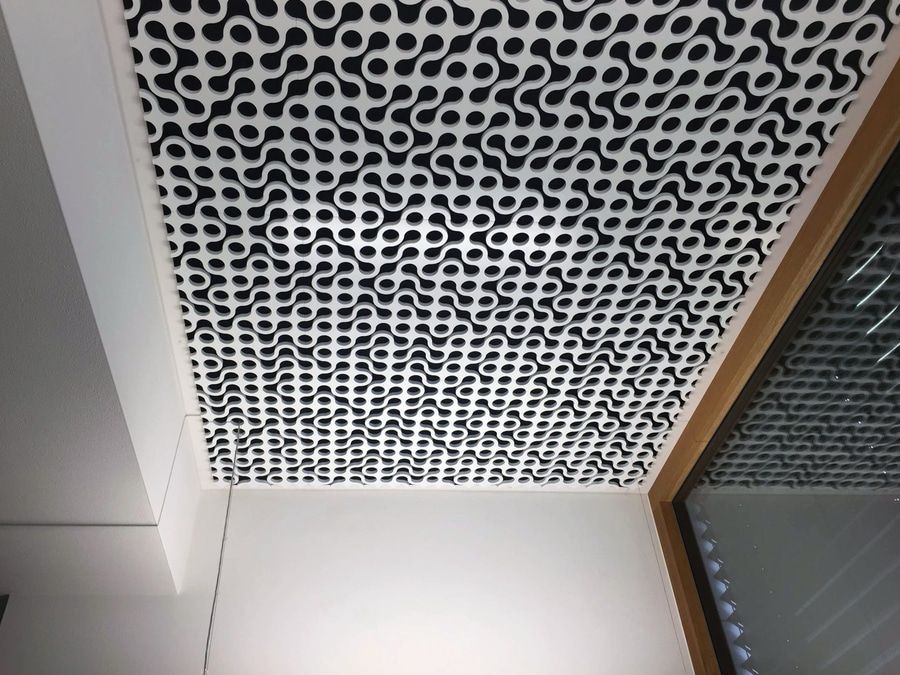This is a photograph taken indoors, capturing a close-up of an intricate metal grate, possibly part of an HVAC system or ventilation cover, mounted on a wall. The grate features a wavy pattern with multiple irregularly shaped holes merging together in an almost abstract design, resembling joined teardrops with varying points of intersection. The metal appears grey and silver, with a blend of black showing through the cut-outs, creating a striking contrast. On the right side of the image, there is a wooden frame, perhaps part of a sliding door with glass panes, and a reflection of the grill is visible in the darker grey. To the left, part of a column or beam covered in sheetrock is seen, adding structural context to the image. At the bottom of the photo, you can see the tiles of the floor, further grounding the setting within the room.